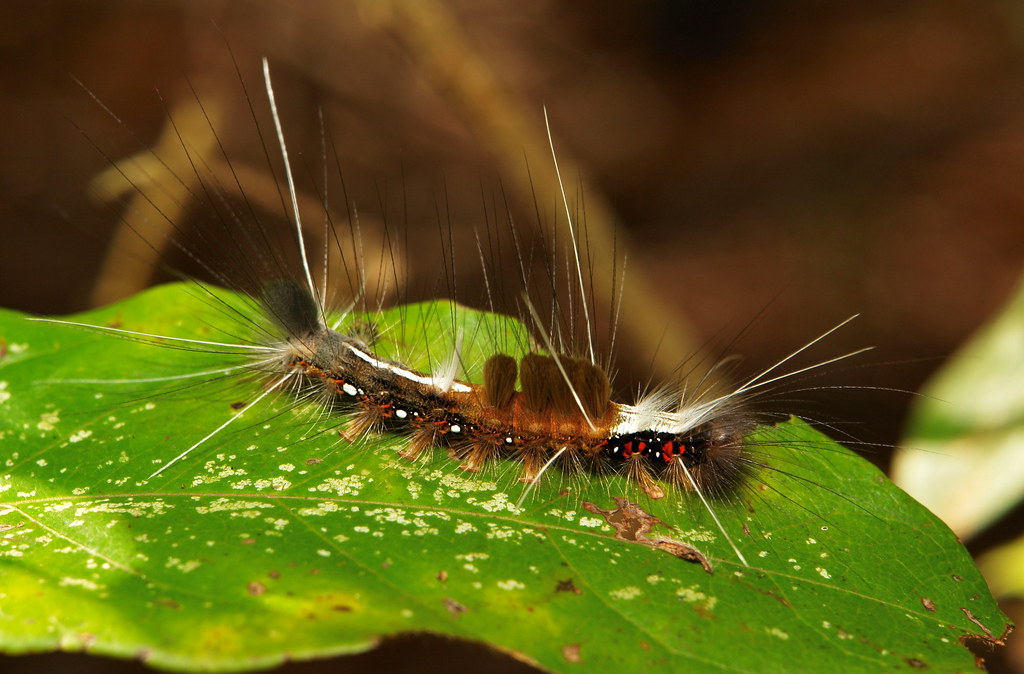The photograph presents an outdoor close-up of a mature, highly detailed caterpillar, centered on a green, veined leaf that's been partially eaten, exhibiting pest damage with brown spots and some fungal-like white spots. The image, wider than it is tall, features a caterpillar characterized by its strikingly diverse and pronounced hairy spines. 

The caterpillar’s body is primarily black with prominent red spots on each segmented section, augmented by brown, white, and black hairy filaments. Notably, the upper part of its back displays four large, vertical brown and white spines, nearly as long as the caterpillar itself, with additional shorter spines on the lower half.

Its intricate coloration includes a white strip running along its back, amidst a mix of long, black and white hairs, resembling the texture of paintbrush bristles. 

The caterpillar’s profile view reveals it is about 6 to 7 centimeters long, crawling from left to right on the leaf. The image background is a blurred brown, likely depicting out-of-focus natural elements such as twigs or leaves, adding to the overall emphasis on the caterpillar and its immediate setting. The detailed capture of the caterpillar’s texture and the leaf’s condition underscores the image's rich, naturalistic quality.